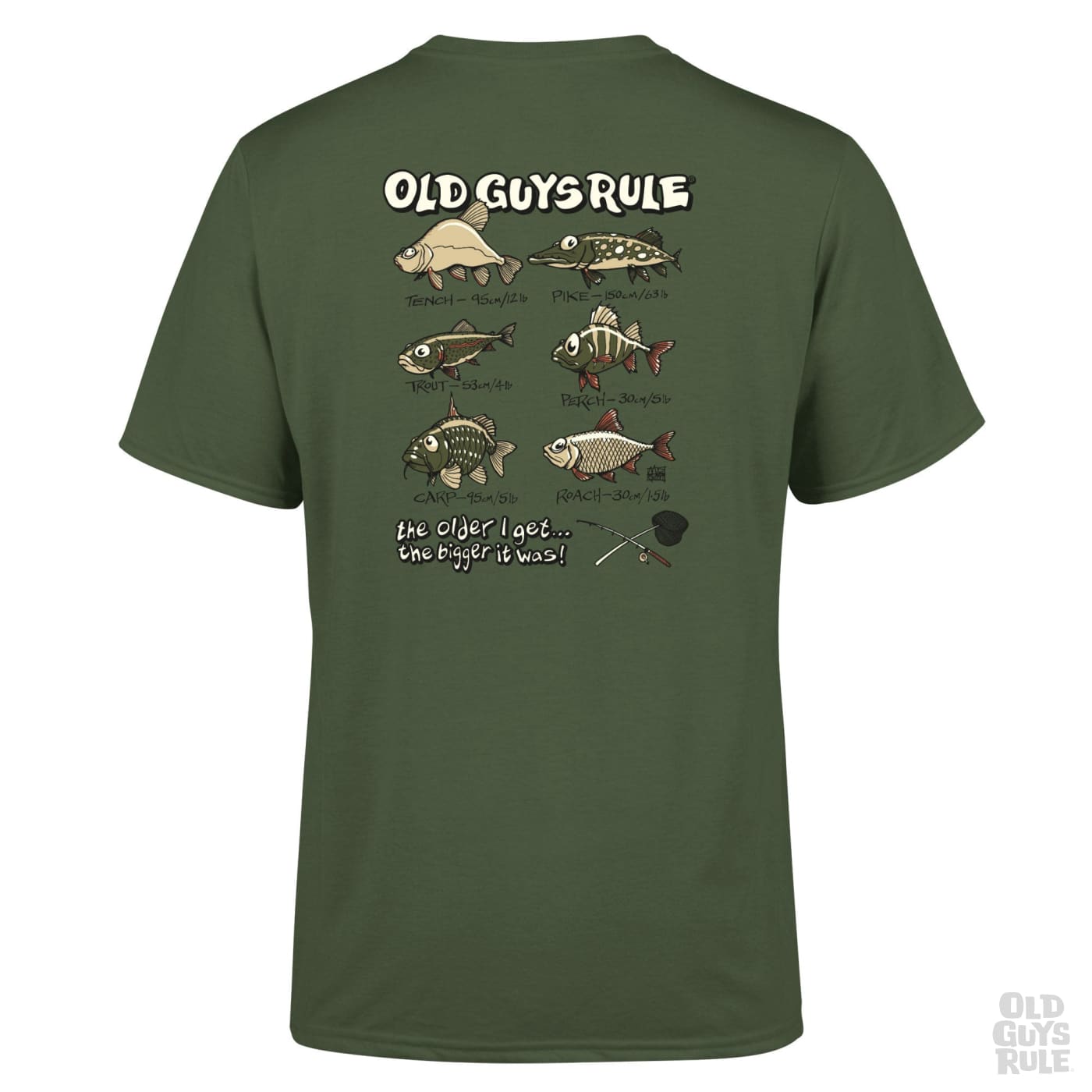This image features a men's olive green t-shirt with a detailed fishing theme. At the top center, the phrase "OLD GUYS RULE" is prominently displayed in bold white uppercase letters. Beneath this slogan, a series of cartoon graphics depict six different fish, each labeled with its name and hypothetical size and weight. The fish include a Tench, Pike, Trout, Perch, Carp, and Roach, each artistically illustrated with various colors such as green, white, red, and black. Below the fish, the humorous caption "The older I get... the bigger it was!" is written in the same white font, adding a playful touch to the design. Complementing the fish illustrations, two fishing poles are crossed like an X on the right side of the shirt; one is decorated with a wind-up reel and the other appears to have a tackle box or hat hanging from the end. The t-shirt combines shades of green, white, brown, and black, creating a cohesive angler's aesthetic perfect for fishing enthusiasts.